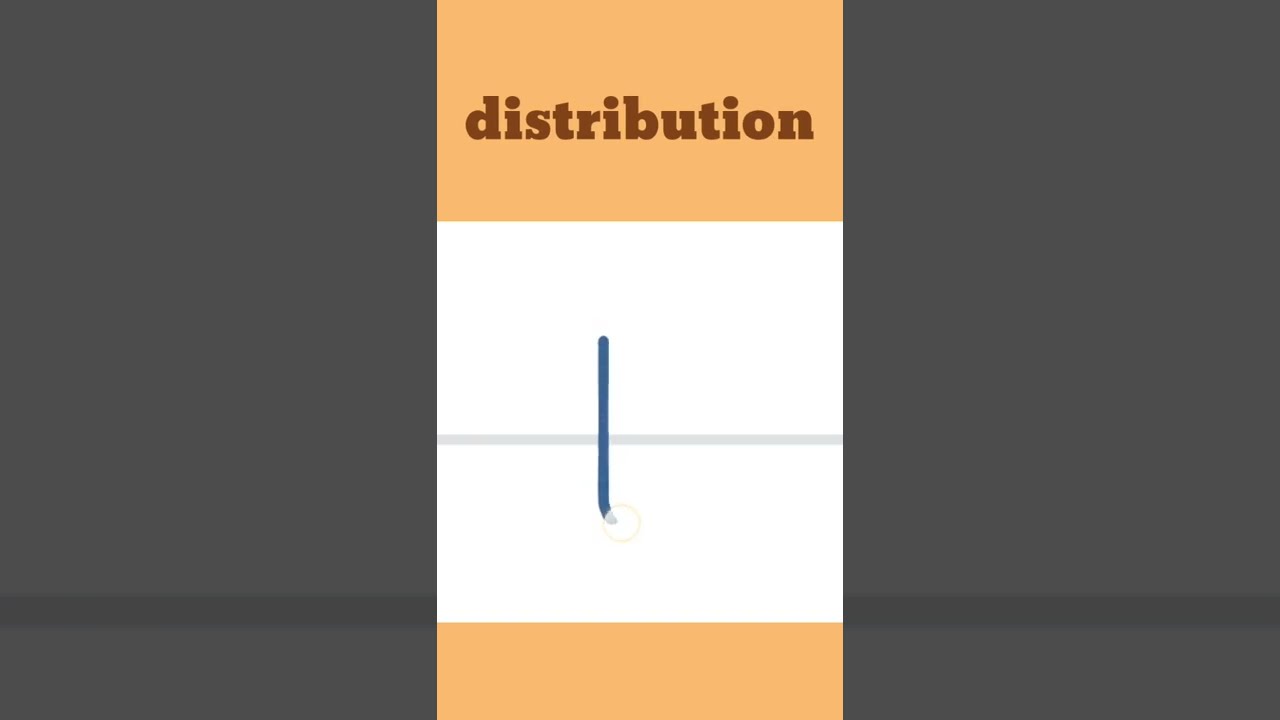The image depicts what appears to be a book cover titled "distribution." The cover is vertically oriented with a rectangular shape. At the top, there is a light orange strip featuring the word "distribution" in small, brown lowercase letters. Below this strip is a white section, which contains a diagram consisting of a horizontal faded blue line intersected at a 90-degree angle by a prominent blue vertical line positioned about 40% from the left edge. The bottom end of this vertical line curves slightly and is encircled by a yellow circle. Beneath this diagram-bearing white section is another light orange strip, which is blank. The background for the rest of the cover is gray, with dark horizontal lines adding a subtle texture at the bottom part.